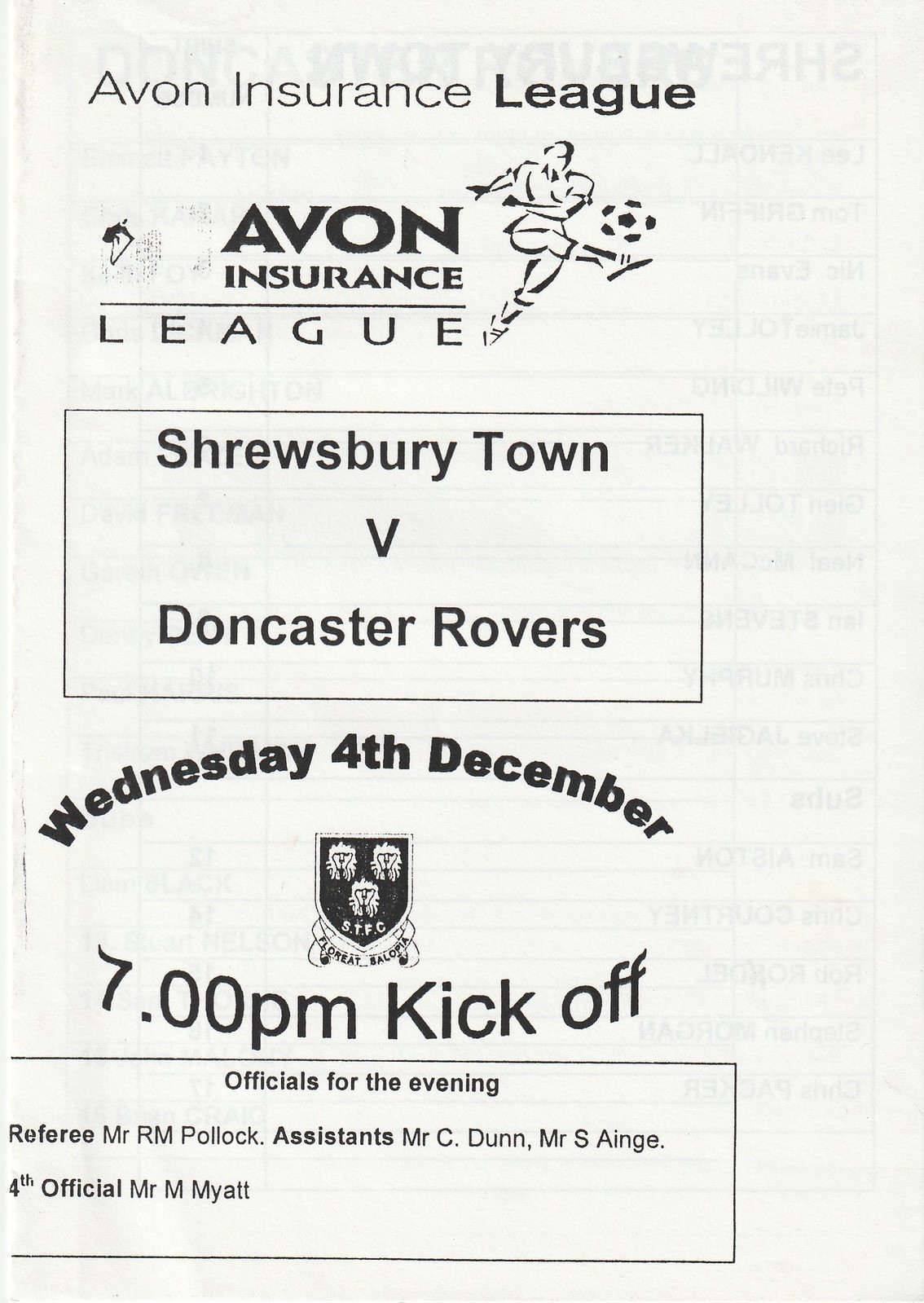The image showcases a sports pamphlet for a soccer game, prominently featuring the text "Avon Insurance League" at the top in a serif font. Below this, the Avon Insurance League logo appears again, accompanied by a stylized illustration of a person kicking a soccer ball. Central to the cover, a black-bordered rectangle states, "Shrewsbury Town v. Doncaster Rovers," with the details "Wednesday, 4th December, 7pm kickoff" positioned just below. Separating this information, a dark-colored shield contains indistinct figures, possibly lions or diamonds, along with the letters STFC. At the bottom of the pamphlet, a section labeled "Officials for the Evening" lists the referee as Mr. R. M. Pollock, with assistants Mr. C. Dunn and Mr. S. Ainge, and the fourth official, Mr. M. Myatt. The back of the pamphlet faintly shows a grid, likely outlining team lineups or game schedules, slightly visible through the paper.